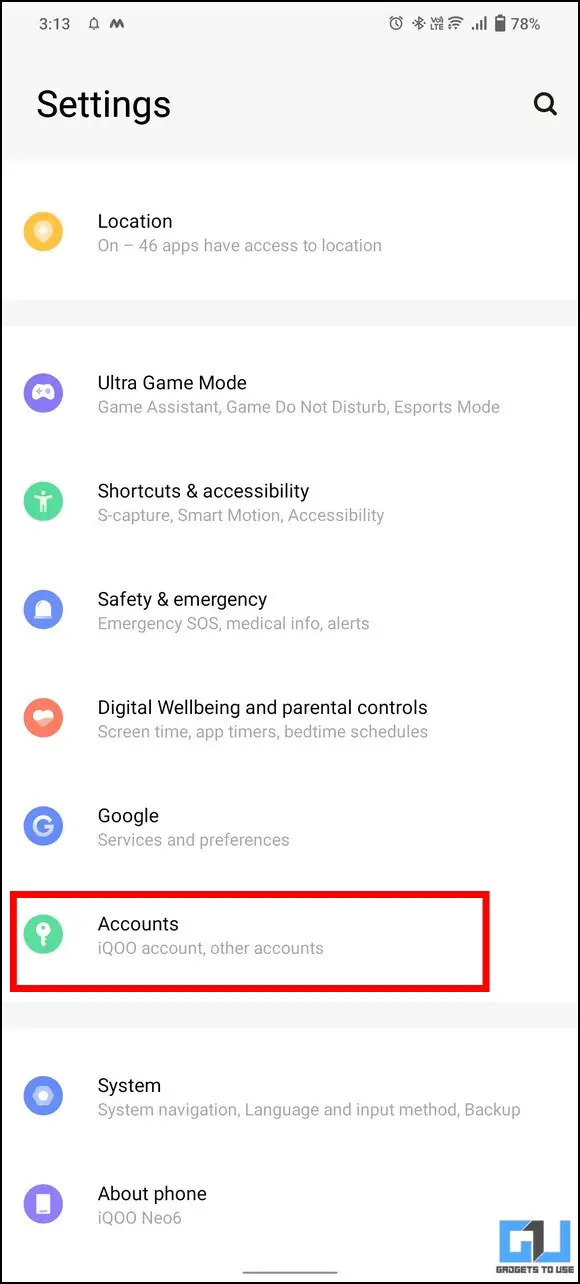Certainly! Here’s a cleaned-up and detailed caption for the image:

---

Screenshot from a mobile phone’s settings page, showcasing a vertical list of circular, color-coded icons. Each icon represents different system settings and is accompanied by descriptive text to the right. The list is organized into sections separated by thin, gray rectangular dividers. At the top, a yellow icon labeled "Location" indicates that 46 apps have access to the user's location. Below it, a purple icon labeled "Ultra Game Mode" includes options such as Game Assistant, Game Do Not Disturb, and eSports Mode. Further down, a green icon labeled "Shortcuts and Accessibility" precedes a blue icon for "Safety and Emergency." The sequence continues with an orange icon for "Digital Well-being and Parental Controls," a blue icon for "Google," a green icon symbolizing "Accounts" marked by a red rectangle, another blue icon for "Systems," and concludes with a purple icon labeled "About Phone."

---